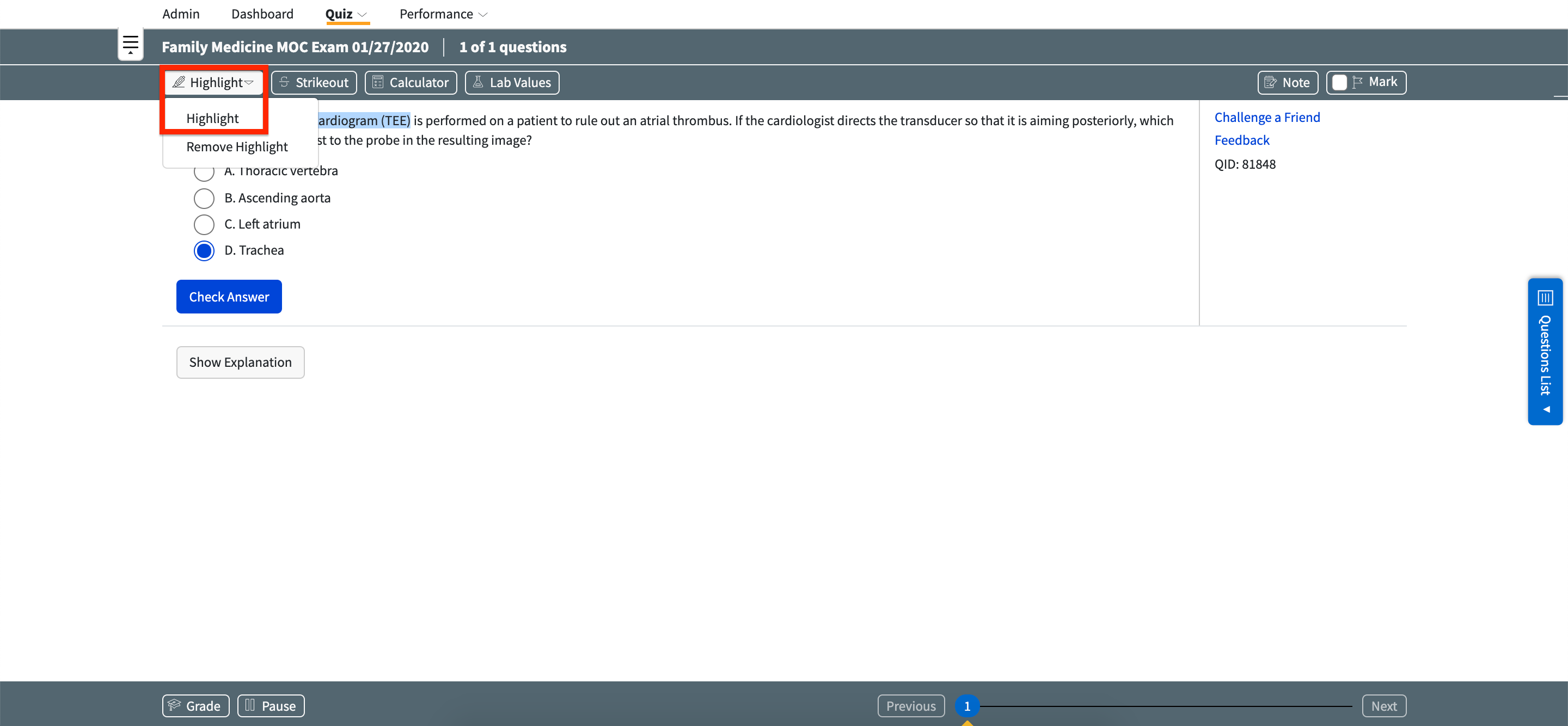Here's a cleaned-up and detailed caption for the image described:

---

The image depicts a webpage, most likely a component of an online platform, dedicated to taking quizzes or exams. At the very top of the interface, the menu displays options labeled as "Admin," "Dashboard," "Quiz," and "Performance." Directly below the menu, a prominent banner indicates the subject as "Family Medicine MOC Exam," dated January 27, 2020. Several interactive buttons are situated beneath this banner: "Highlight," "Strikeout," "Calculator," and "Load Values," with additional buttons labeled "Note" and "Mark" positioned on the right side.

The "Highlight" feature appears to be active, as evidenced by the dropdown menu below it, although the content within this dropdown is difficult to decipher. Below this section, the exam question is presented in a multiple-choice format with options labeled A, B, C, and D. The user has selected option D, which contains the word "crackier." 

Further down the page, there are buttons labeled "Check Answer" and "Show Explanation." The lower portion of the page appears largely blank, save for a sidebar on the right that lists options including "Questions List," "Challenge a Friend," and "Feedback," accompanied by a feedback code.

---